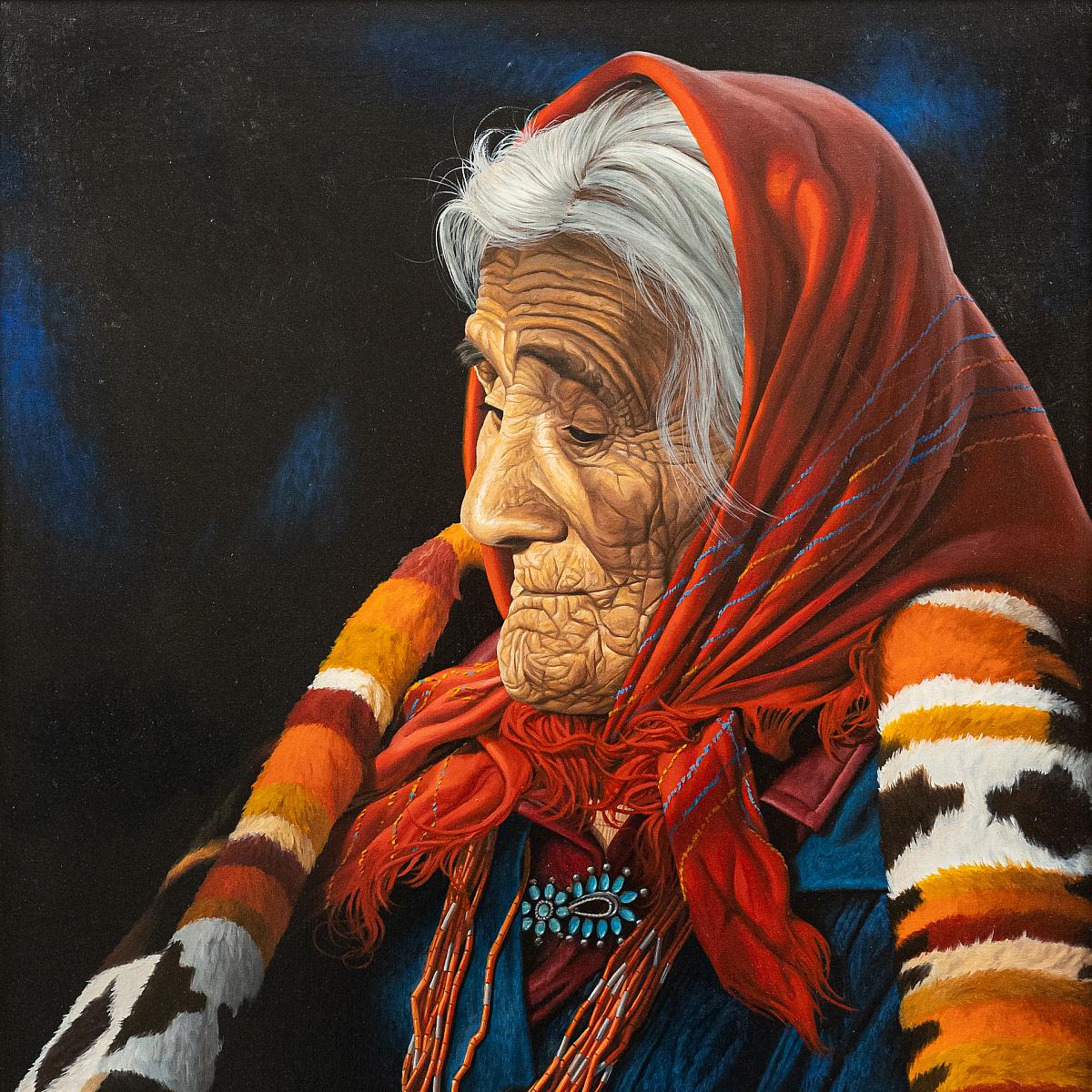This artwork depicts an elderly Native American woman captured in a highly detailed illustration. Her face, deeply etched with age, is a tapestry of wrinkles, especially pronounced on her forehead and chin, giving her tanned, leathery skin a striking texture. The woman’s white hair peeks from beneath a vibrant red babushka or scarf draped around her head. A richly colored blanket, adorned with tribal patterns in hues of oranges, burgundies, browns, yellows, whites, reds, and blacks, wraps around her shoulders. She is also dressed in a blue coat over a burgundy blouse, which is fastened at the neck by a decorative clasp. Around her neck, she wears a striking necklace featuring turquoise and numerous orange beads. The background of the piece is dark, possibly indicating a nighttime setting, further emphasizing the rich colors of her attire and the intricate details of her venerable visage.